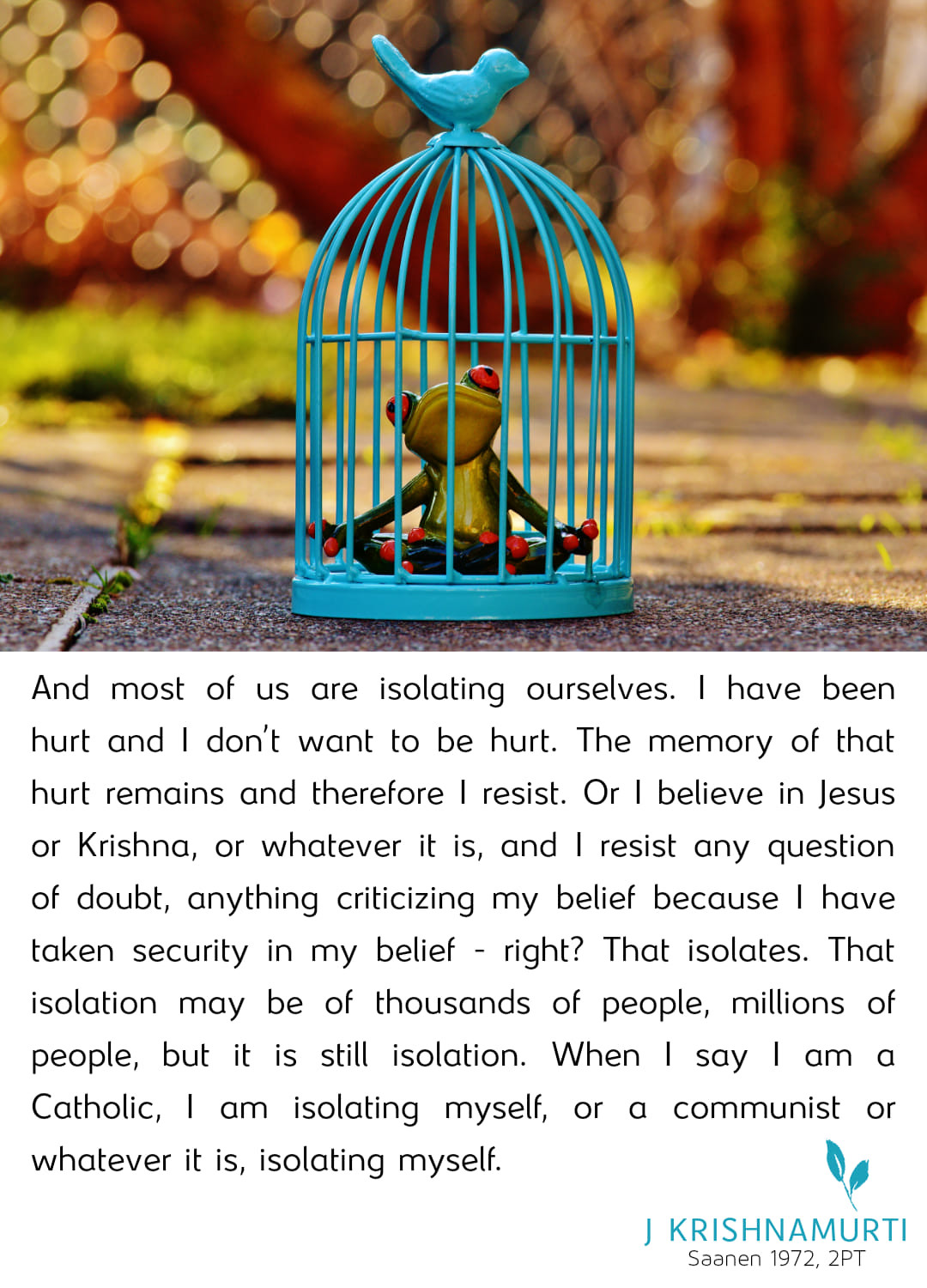The image is a close-up, rectangular photograph taken outdoors, featuring a small aqua blue birdcage positioned in the center, resting on a pavement. The background is blurred, showcasing vague hints of brown, red, and green, possibly indicating tufts of grass emerging from the ground. Within the intricately designed birdcage, complete with a blue bird perched on the top, sits a toy frog figurine. This frog has large, striking orange eyes and a green body with a yellow chest, alongside red fingers and toes. The frog's eyes appear to be directed towards the camera. The bottom half of the image transitions to a white background with black text, containing a profound quote attributed to J. Krishnamurti from 1972. The quote discusses themes of isolation due to hurt and belief, ending with a mention of isolating identities such as being a Catholic or communist. Below this, in the lower right-hand corner, there is an image of a blue twig with two leaves, accompanied by the name "J. Krishnamurti" in blue text and the inscription "Sanen 1972 2PT."